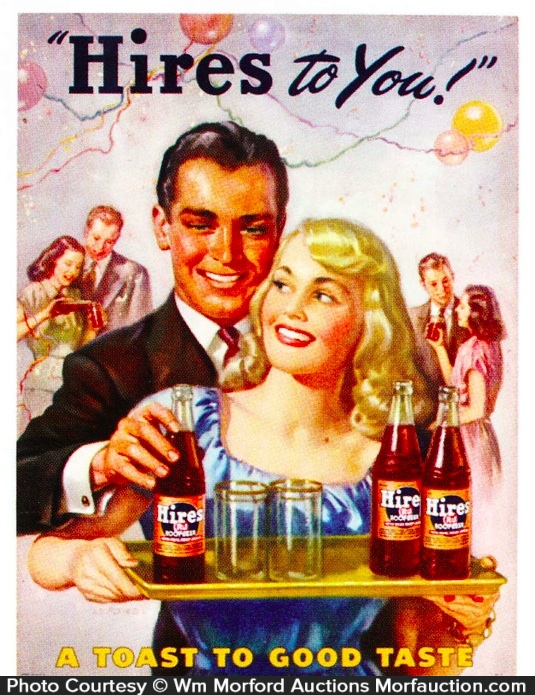This is an image of a vintage advertisement for Heyer's Root Beer, likely from the 1950s or 60s. The ad is centered around a lively party scene with the slogan "Heyer's to you" displayed at the top in black, decorative text, with "Heyer's" in a distinctive font and "to you" in cursive italics. In the foreground, a strikingly handsome couple is featured: a blonde woman in a blue dress holding a golden yellow tray, and a man in a suit and tie standing directly behind her, appearing to reach for a bottle. The tray holds three bottles of Heyer's Root Beer and two empty glasses ready to be filled. The background depicts two additional couples, celebrating amidst balloons in shades of pink, orange, white, and yellow. The overall scene is imbued with a festive atmosphere, accentuated by streamers and jubilant expressions. The advertisement concludes with a yellow text at the bottom stating, "A toast to good taste," followed by a black strip that reads, "Photo courtesy, copyright W.M. Morford Auctions, morauction.com."